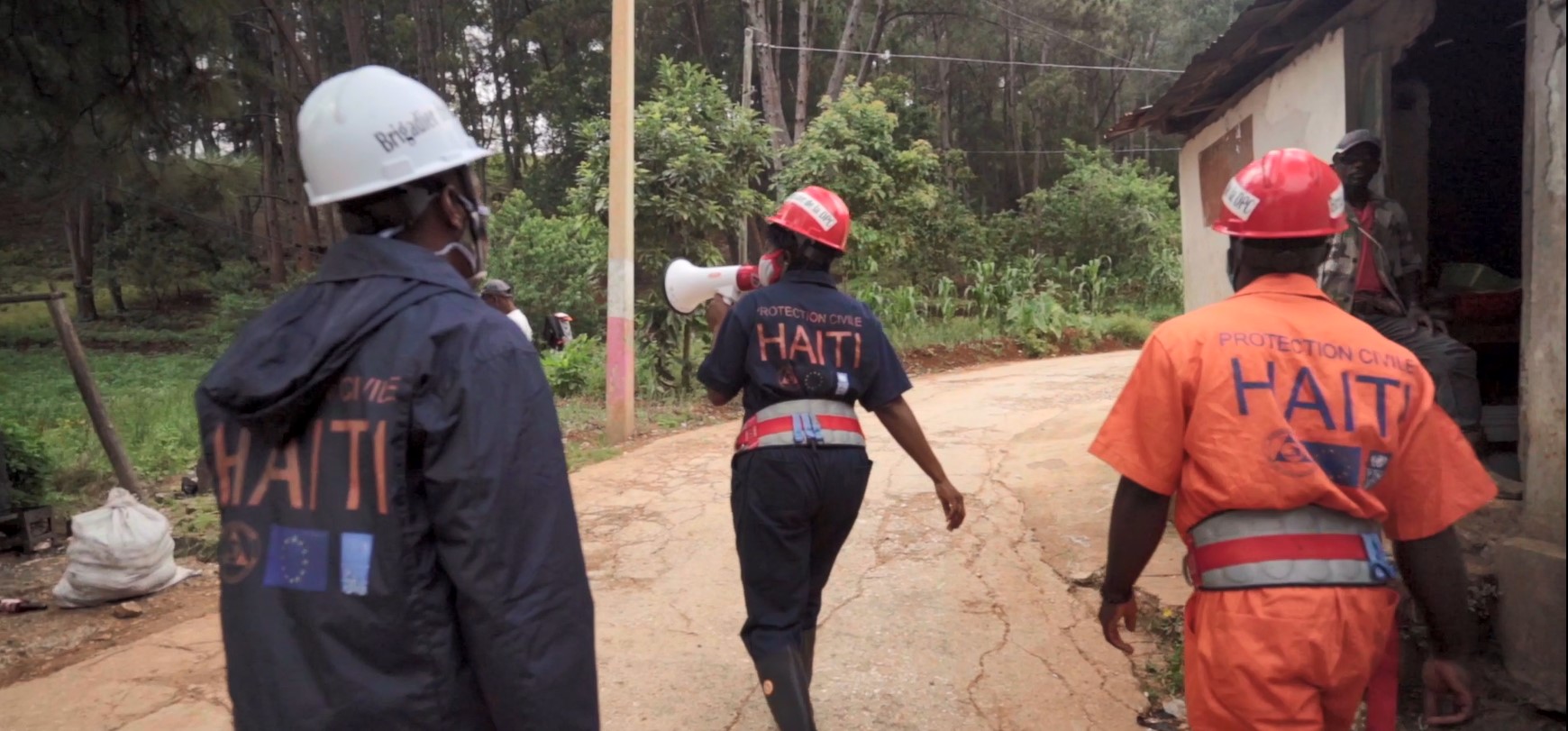In this outdoor photograph, three workers are walking away along a cracked, beige stone pathway set in a lush jungle area. Dominated by greenery and tree trunks on the left, a white building with a person in the doorway stands on the right side of the image. The workers' matching outfits display "Protection Civil Haiti" on their backs, adorned with a series of symbols. Central among them is a woman wearing a dark jumpsuit with orange lettering, an orange hard hat, a face mask, and slightly darker matching boots, holding a white megaphone. To her left, a man is dressed in a dark blue jacket with the same orange lettering and a white hard hat. On her right, another man sports an orange jumpsuit with blue lettering and an orange hard hat.